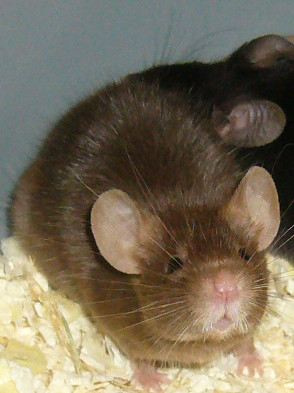A close-up photograph features a small, active brown-furred mouse with beige-colored ears on their interior. The mouse has a pink nose and pink-colored paws, nestling amongst light yellow-colored wood shavings in a cage. With its beady black eyes and long whiskers, the mouse appears fully alert and engaged, staring directly at the camera. Notably, the mouse's fur is fairly long on its back, and a second mouse, possibly of the same breed, is slightly obscured in the background. The wood shavings and setting suggest a comfortable and familiar environment for the rodents.